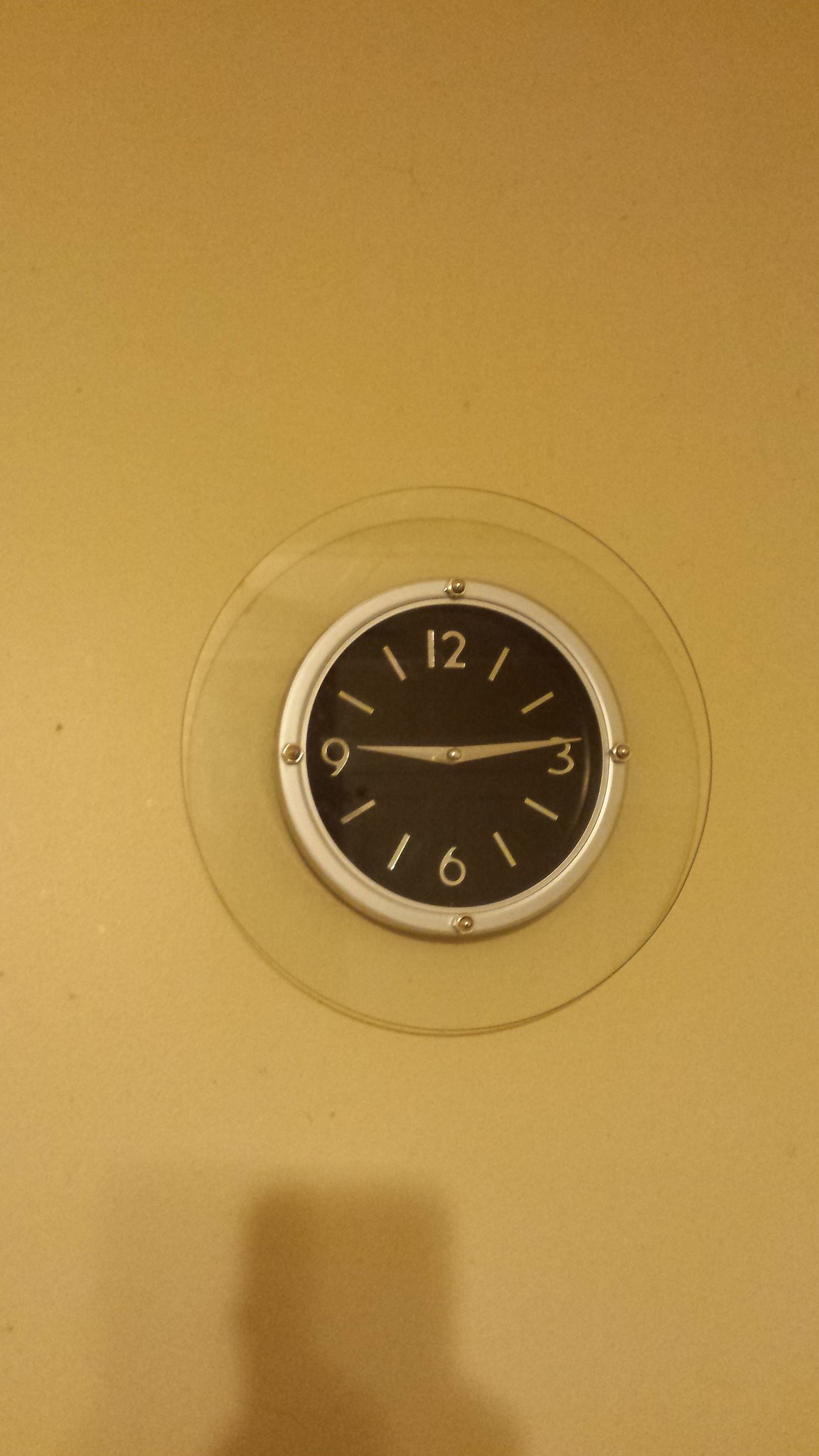The image, in portrait orientation, captures a wall clock mounted on a yellow wall. The clock is circular with a clear, plastic outer frame. Inside this frame, there is a metallic silver rim securing the clock. Four visible screws at the 12, 3, 6, and 9 o’clock positions hold the clock face in place. The clock's face is black, featuring silver-aluminum numbers at the 12, 3, 6, and 9-hour marks, with simple lines indicating other hours. The intricate silver hands show the time as 9:15. In the lower part of the photo, the shadow of the photographer’s hand and cell phone is cast on the wall, suggesting they are holding the device in their right hand.